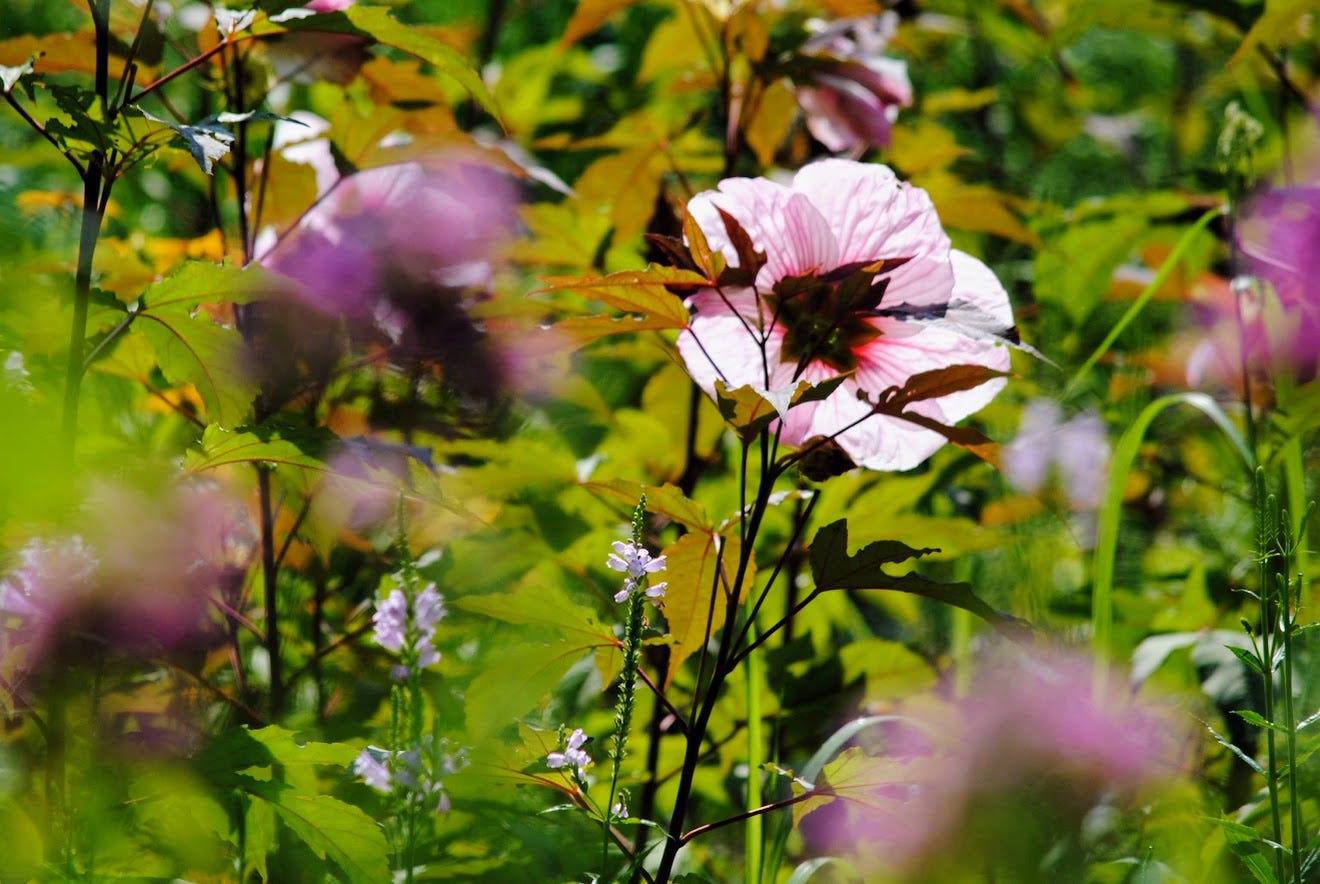This photograph captures a close-up view of various flowers in a dense, wild field. Dominating the right center of the image is a single, sharply-focused bloom with light pink petals and a dark purple center. Surrounding this main flower are at least five other blooms, which are slightly out of focus and share similar light pink coloring. Interspersed among the flowers, there are tall green stems and leaves, some displaying a yellow to orange hue. Additionally, scattered throughout the scene are a few white dandelion-like blossoms. The background is a blend of darker-colored stems, green leaves, and blurred petals, suggesting the photograph was taken in natural sunlight during the day. The overall composition evokes the sense of a wild, unmanicured flower field teeming with life.